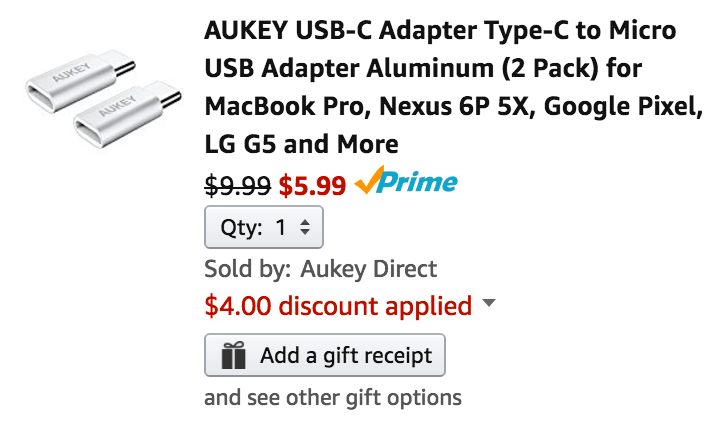The image is a screenshot of a product page on the Amazon shopping website, showcasing two USB adapters positioned on the left side of the screen. These adapters, each featuring a white plastic body, are branded with "AUKEY" written prominently on their surfaces. To the right of the adapters, the product details are displayed in black text: "AUKEY USB-C Adapter. Type-C to Micro USB Adapter. Aluminum, 2-Pack for MacBook Pro, Nexus 6P/5X, Google Pixel, LG G5 and more." Below this descriptive text, the original price of $9.99, written in black, is crossed out with a horizontal line. Adjacent to the original price, the discounted price of $5.99 is indicated in red.